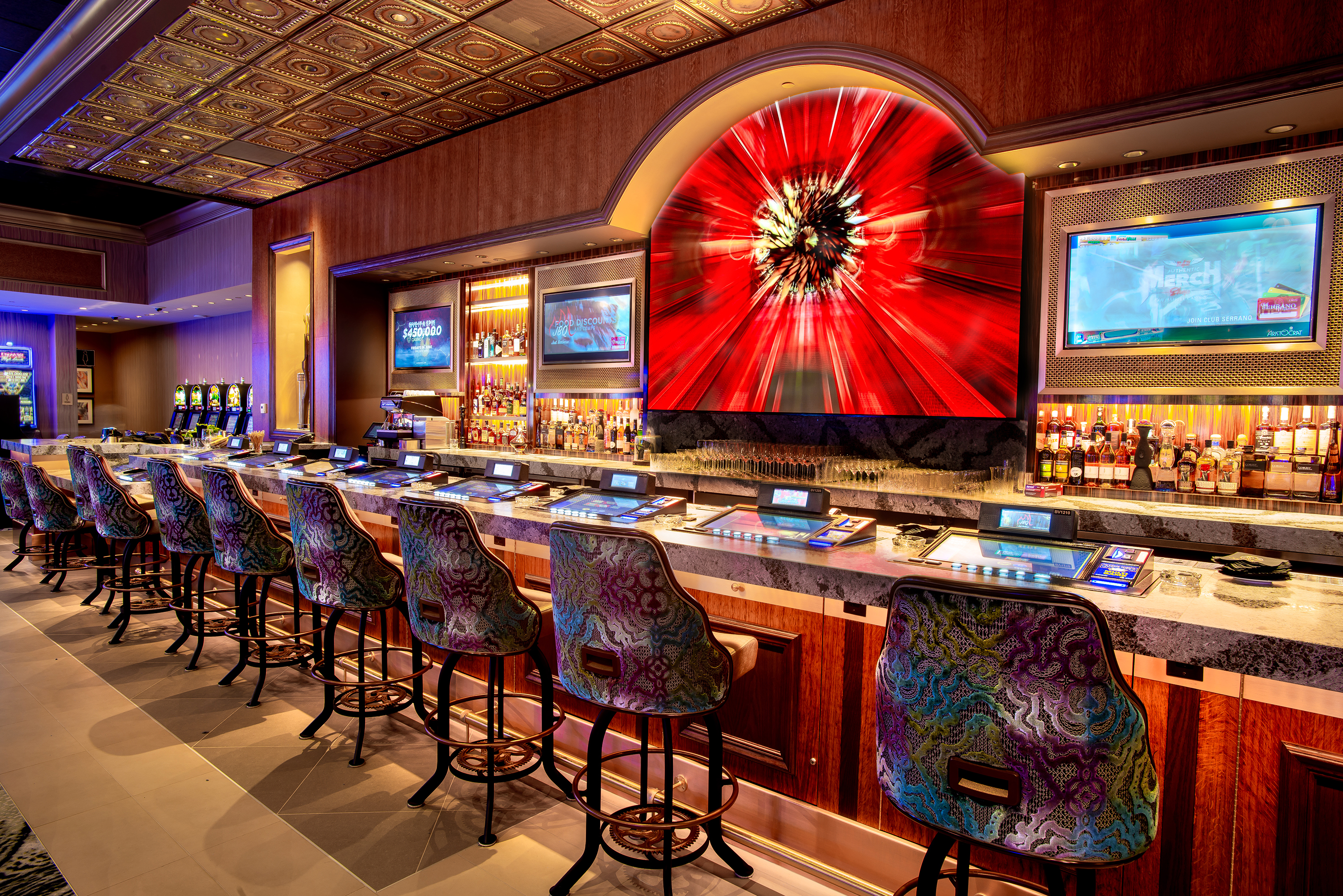This photograph captures the vibrant interior of a casino bar. In the foreground, ten bar stools with colorful, multi-hued backs in shades of purple, green, blue, mauve, gold, and white are neatly lined up. Each stool has a wrought iron base, adding to the bar’s stylish decor. The bar counter features individual gaming screens, resembling small arcade consoles, at each seat. Behind the bar, shelves are filled with a variety of alcoholic bottles. The walls on either side of the bar also display an array of drinks. The centerpiece of the back wall features a striking red design with hints of yellow and gold, surrounded by black accents and a video screen. To the left, several slot machines add to the casino ambiance. The entire space is brightly lit, showcasing the rich wooden panels and the eclectic mix of colors that enhance the lively and luxurious atmosphere of the casino bar.